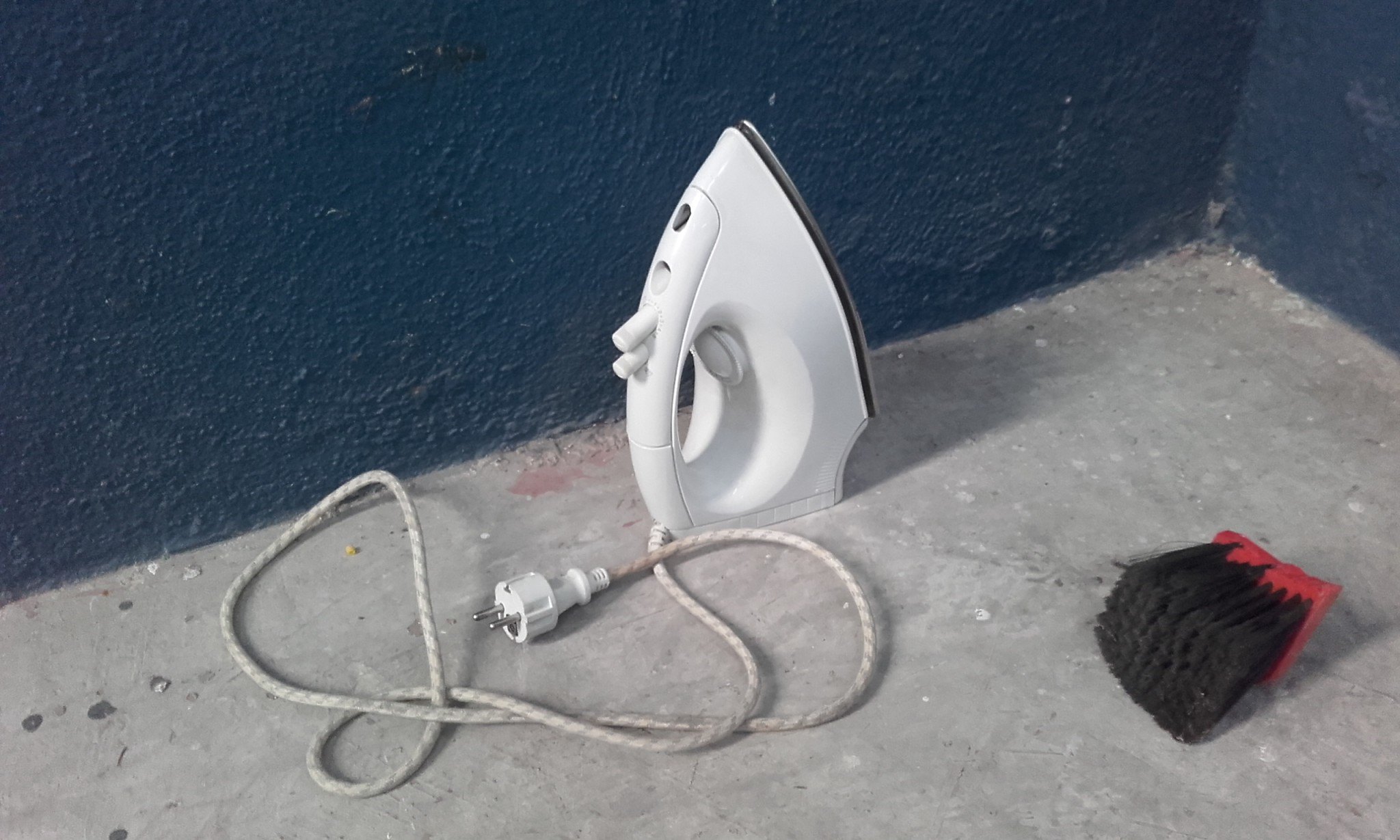This photo captures a scene set against a weathered, dark navy blue stucco wall, showcasing a rectangular red brush with black bristles lying on a gray concrete floor. Adjacent to the brush is a white clothing iron with a silver ironing plate, standing upright on its base. The iron features two push buttons on the handle and a white braided cord with gray stripes extending from its back, ending in a European-style plug. Behind these objects, the textured wall shows signs of age and weathering, adding a vintage feel to the image.